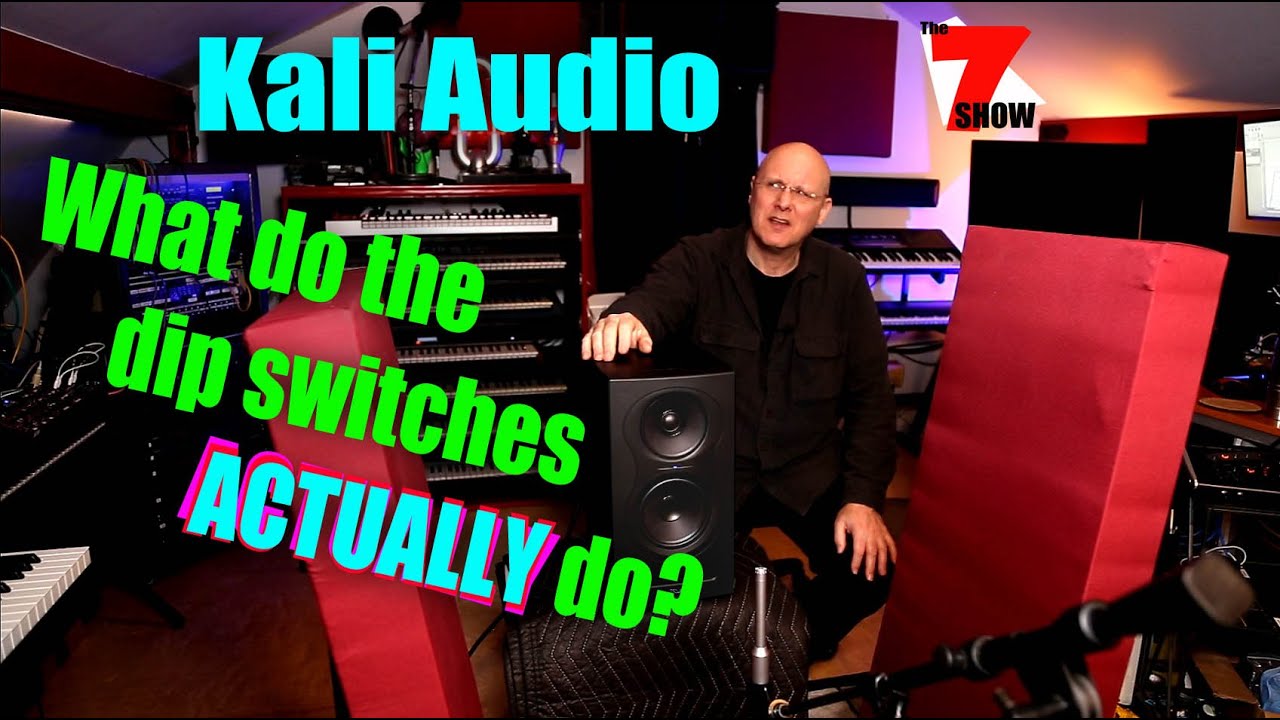The digital advertisement in the horizontal rectangular image presents an older, bald white man with glasses, wearing a black long-sleeved button-down shirt over a black t-shirt, paired with black pants. He sits in a cluttered studio with white walls, surrounded by various electric keyboards, plug-in analog synthesizers, and a microphone at the bottom right. The man is seated on an indistinguishable surface with one hand propped up on a vertical, rectangular black speaker featuring two large speaker cones. His other hand rests on his knee as he gazes forward with a slight smile. The top left corner of the image displays the text "Kali Audio" in blue letters, with the caption "What do the dip switches actually do?" below it in bright green, featuring the word "actually" highlighted in light blue with a pink border.